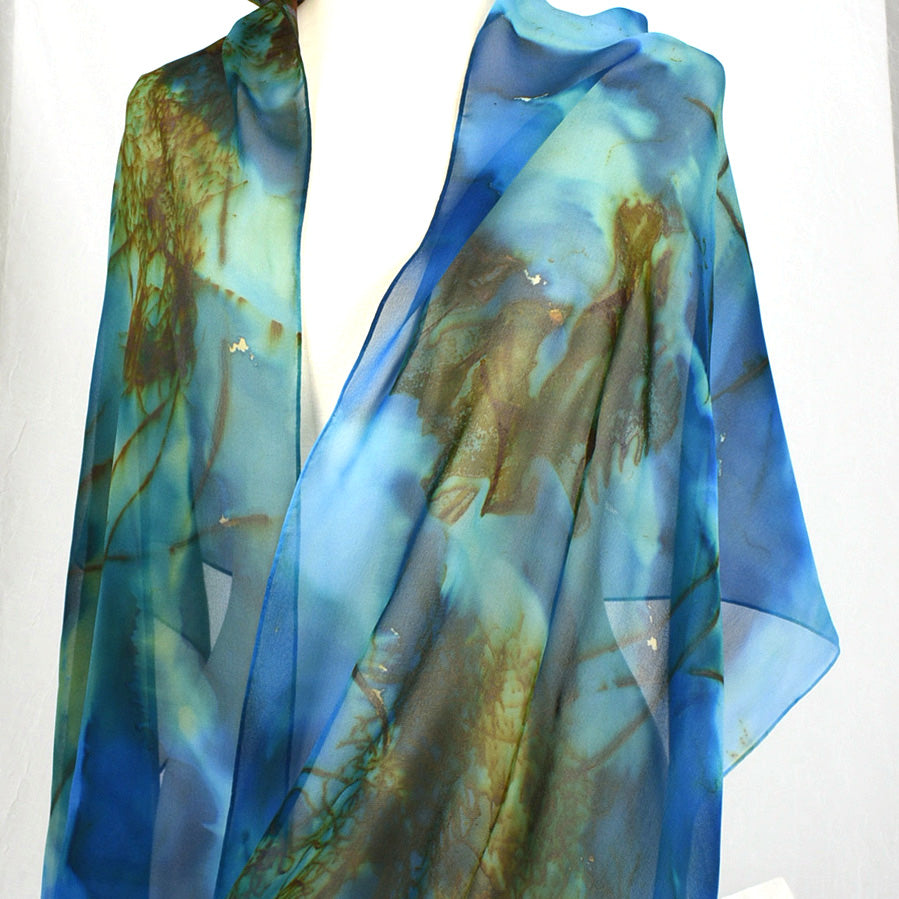The photograph features a long, flowing shawl draped against a white background, likely on a mannequin, emphasizing its translucent and almost ethereal quality. The shawl, designed in various shades of blue, ranging from light blue to navy, and accented with teal, features intricate brown and green decorations that resemble plants or straw, evoking a watercolor effect reminiscent of nature scenes such as the ocean and earth. The V-shaped neckline, combined with its loose, wavy fit, suggests it can be worn as a shawl, scarf, or headscarf. The overall presentation appears to be an advertisement, possibly for a secondhand or online marketplace.